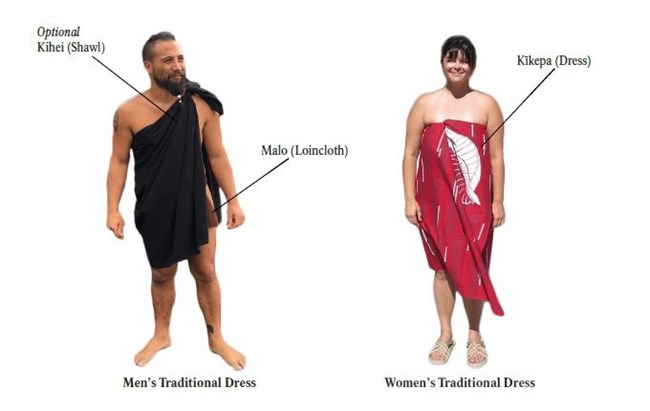This image depicts a man and a woman, both of average age and height, adorned in traditional Islander apparel. The man, positioned on the left, is sporting a beard and mustache with a partially shaved head. His attire includes a black sashed robe called an optional kihei or shawl, and a malo or loincloth around his pelvis. He is barefoot and smiling, looking slightly to his left. Text in the image labels his attire as "men's traditional dress."

The woman on the right is smiling directly at the camera. She is wearing sandals and a red robe, referred to as a kikapa or dress. Her shoulders are exposed, and her dark, short hair frames her face. The text next to her describes her outfit as "women's traditional dress." Both individuals exude a sense of cultural pride, with their traditional garments and the clear, informative labels providing insight into their native attire.